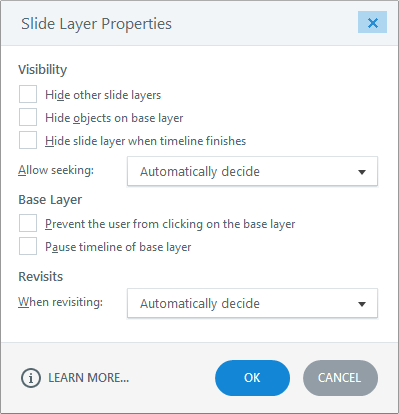The image depicts a section of settings labeled "Slide Layer Properties." This section is presented in a compact dialog box that occupies the center of the screen. In the top right corner, there are two prominent buttons: one blue button labeled "OK" and another green button labeled "Cancel."

The main content of the dialog box is divided into several sections, each controlling different aspects of slide layer visibility and behavior. At the top, there is a section titled "Visibility," which includes three checkboxes with the following options:
1. Hide Other Slide Layers
2. Hide Objects on Base Layer
3. Hide Slide Layer When Timeline Finishes

Beneath the "Visibility" section is the "Allow Seeking" field, accompanied by a dropdown menu currently set to "Automatically Decide."

Following this, there’s a section titled "Base Layer." It consists of several options and checkboxes:
1. Prevent the User from Clicking on the Base Layer
2. Pause Timeline of Base Layer

An additional field called "Revisits" appears with the sub-heading "When Revisiting." This is also accompanied by a dropdown menu set to "Automatically Decide."

At the bottom of the dialog box, there's a clickable link labeled "Learn More," presumably to provide further information or assistance on configuring these properties.

Overall, the detailed settings in this dialog box offer a range of customizations for managing slide layers, visibility, and user interactions within a presentation or e-learning module.